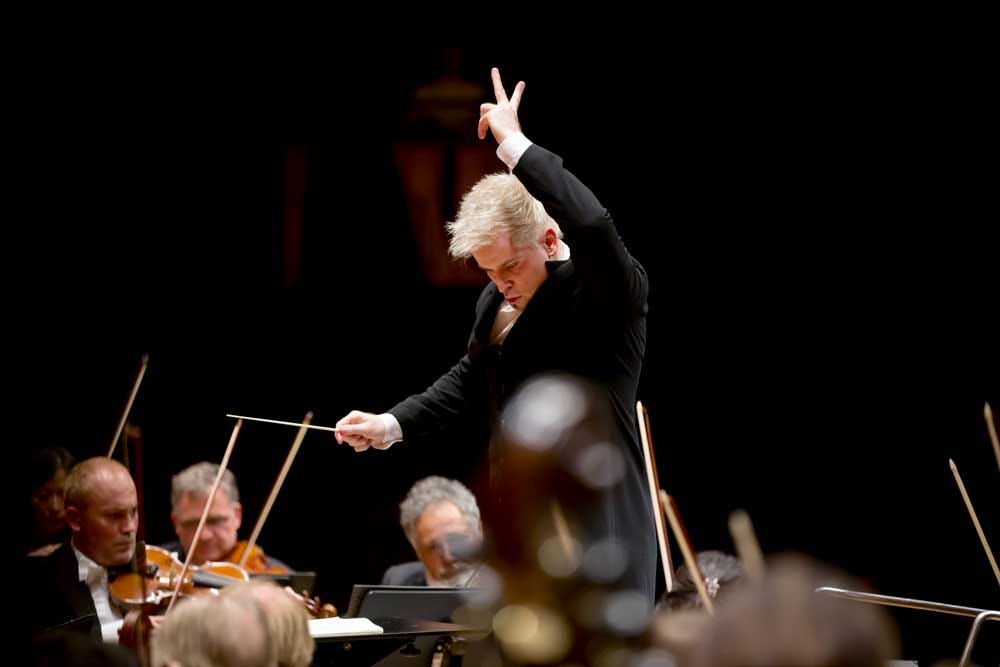This color photograph captures a moment during a classical music concert featuring an orchestra. At the center stands an older Caucasian conductor with gray hair, dressed in a black suit over a white shirt. His left hand is raised with two fingers extended, while his right hand, holding a white baton, is positioned lower. The conductor’s head is slightly lowered, focusing intently on his task. Partly obscuring him in the foreground is a blurred, out-of-focus musical instrument.

Surrounding the conductor, particularly to his lower left, are violinists, identifiable by their protruding bows. These musicians are also dressed in black suits with white shirts. The violinists' music stands are visible to the right. The photograph’s background is entirely black, emphasizing the central figures and adding a dramatic ambiance to this classical musical setting. The image overall depicts a harmonious moment, with the conductor and orchestra immersed in a performance, suggesting a scene filled with movement and focus.